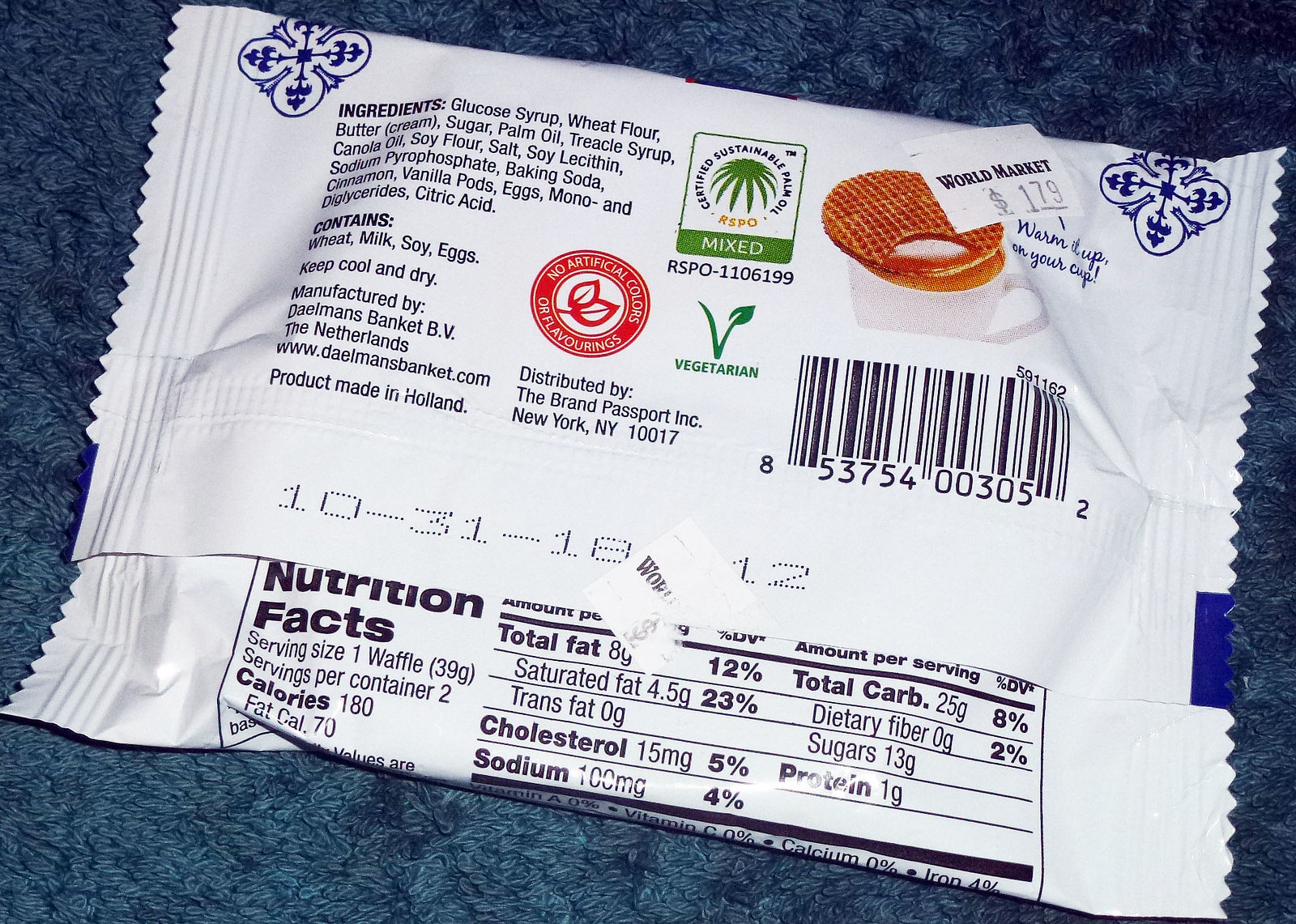This photo showcases the back of a white, rectangular Stroopwafel package adorned with blue decorations. Positioned on a blue, fuzzy surface that could be a towel or carpet, the package prominently features a World Market price tag of $1.79 partially covering an image of a Stroopwafel in the upper right-hand corner. Beside the image, text reads "warming up on your cup." At the middle top, a label indicates "Certified Sustainable Palm Oil, RSPO Mixed," while another label asserts "No artificial colors or flavors" and the package is marked as vegetarian. 

The left side of the package contains detailed ingredients, indicating it includes wheat, milk, soy, and eggs, along with a manufacturer note stating it’s made in the Netherlands. A barcode and an expiration date of 10-31-18 are displayed on the right-hand side, above the partially covered nutritional facts at the bottom. The package also advises to "keep cool and dry."